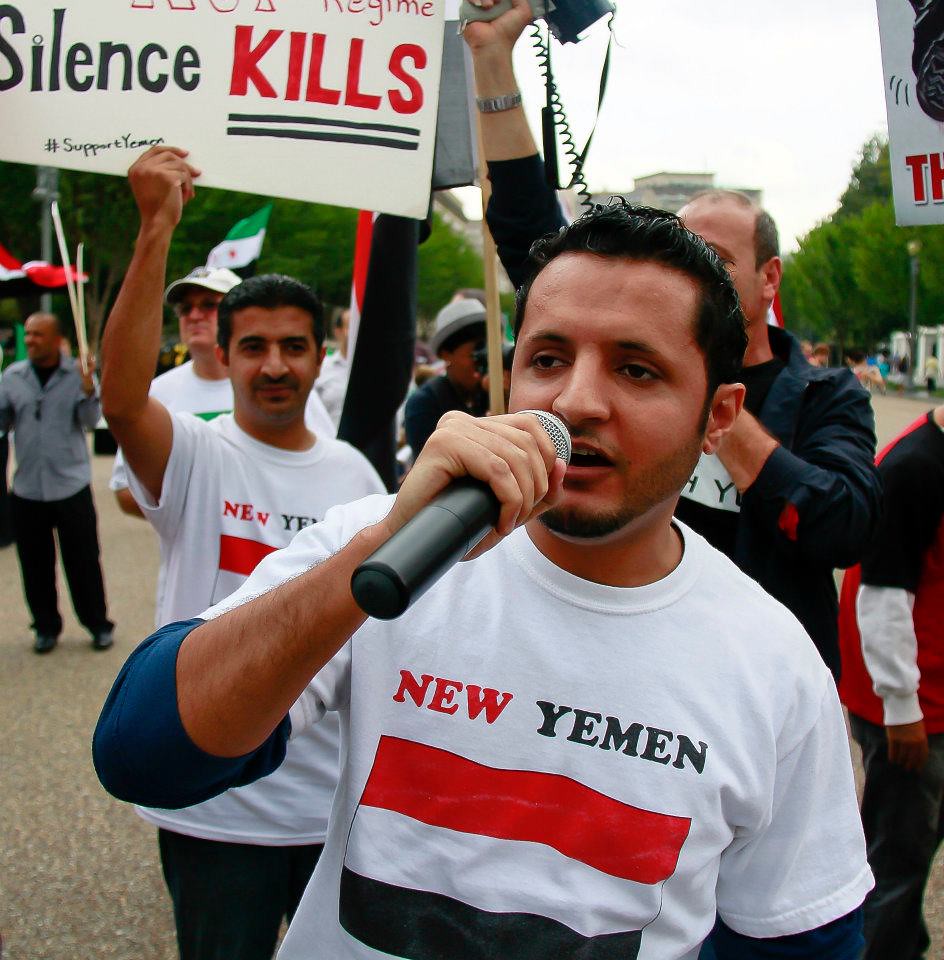The image captures a daytime protest, possibly in Yemen, with the focal point being a man in the foreground. He has dark skin, black hair, and a beard and mustache. He is holding a microphone with his right hand close to his mouth, wearing a long-sleeved blue shirt rolled up to the elbows, with a white short-sleeved t-shirt over it. The t-shirt prominently displays "New Yemen," with "New" in red and "Yemen" in black. The shirt also features a flag with red, white, and black stripes. The protesters are walking down a paved road lined with trees, with some gravel visible on the ground. There are other people in the background also wearing "New Yemen" shirts and different attire. One person is holding a partially visible sign that reads "Silence Kills," with "Kills" in red and underlined twice, followed by the hashtag #SupportYemen. Another individual is seen holding a camera, while a man behind the main speaker is using a bullhorn. The scene appears to be in a capital city, given the presence of large buildings and an overcast sky in the background.